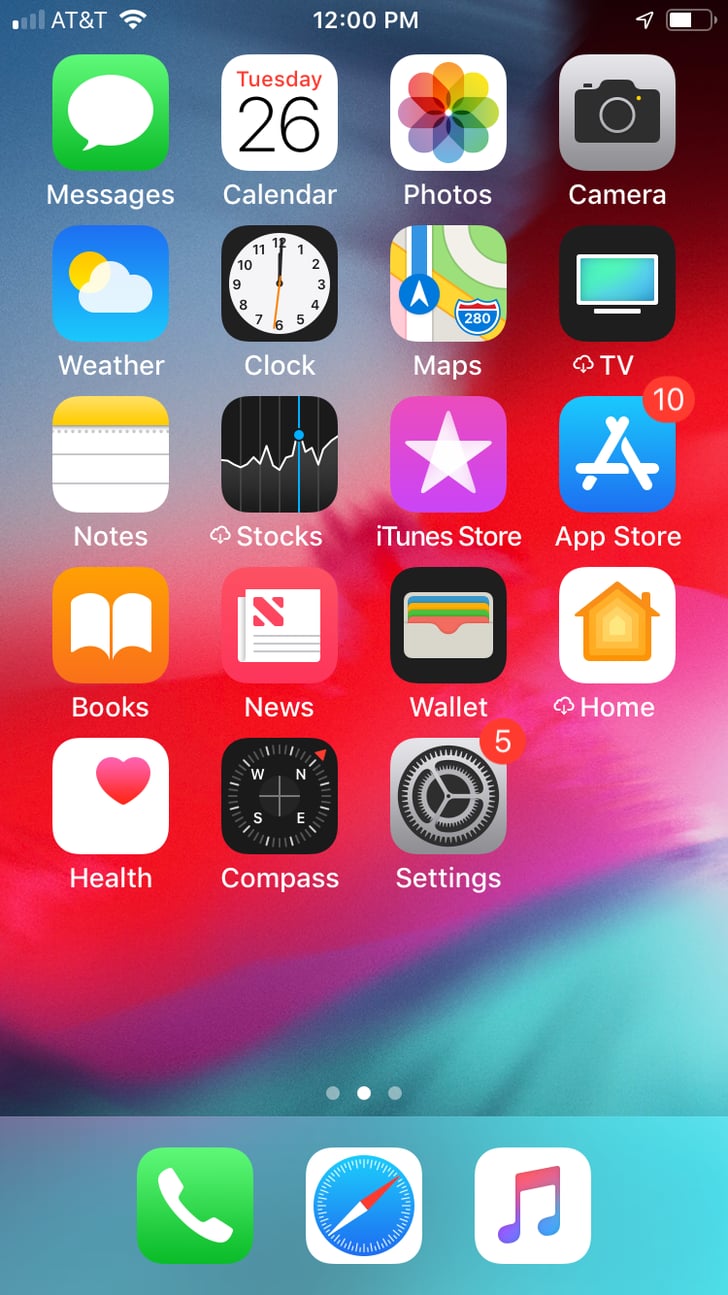The image displays an organized collection of app icons on a vibrant, multi-colored background. 

In the top left corner, there's a green square symbolizing a speech bubble, indicating the messaging app. Adjacent to it lies the calendar app, showing "Tuesday 26th". The photos app stands out with its colorful icon next to a gray square featuring a camera logo.

The weather app is represented by a square showing a cloud and a yellow sun. Below it, there's a clock icon depicting three hands. The maps app is followed by a TV icon, a notepad, and an app with a pair of socks on it.

A thin blue line separates these icons from the rest. Below this line, a purple square with a white star signifies the iTunes Store. The blue app next to it represents the App Store. Icons for books and news appear sequentially, followed by a wallet app icon displaying different types of cards.

A noticeable white square with an orange house in the center represents a home-related app, and another white square showcasing a heart suggests a health or fitness app. The compass app, connected to a star icon, is next to another gray square.

Towards the bottom, a gear icon indicates the settings app, marked with five notifications. To the right, a green square with a white headset represents the music or audio app. Lastly, a white square with a musical note appears, likely representing a music app. 

This detailed arrangement of app icons is set against a vividly multi-colored background.